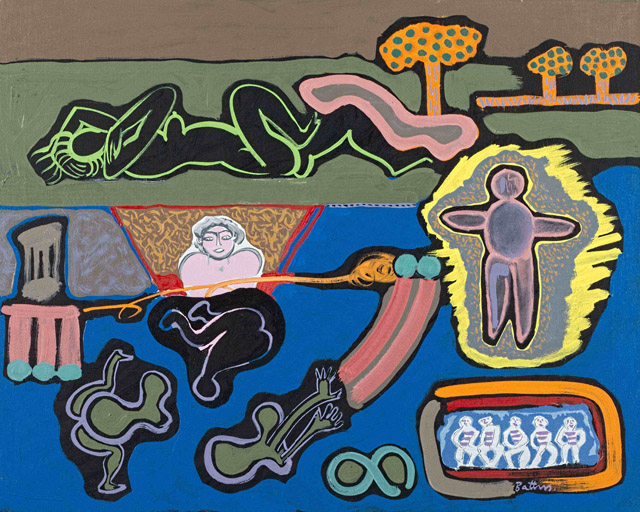The painting features a surreal composition divided into three horizontal bands. The topmost narrow band is brown, while the striking green band beneath it depicts a cartoon-like profile of a naked woman, her breasts exposed. This green segment is populated by three whimsical orange trees adorned with green polka dots. A pink blob touches the woman’s knee and leg, enhancing the playful yet enigmatic scene.

Below this, in the blue band, a series of unusual and intriguing figures emerge from the blue background. To the left, a gray structure with black splotches stands prominently. Next to it, a pink structure with three vertical bands, tipped in green, ascends, while an inverted triangle forms another surreal female figure, clad in pink and wearing glasses, visible only from the waist up. Below her, an upside-down child seems to be in the process of being born.

Flanking this central action are two green body-like blobs. One of these green forms extends into an orange curved structure ending in two blue spheres. To the right of these spheres, a cruciform person outlined in gray and yellow appears, their arms, legs, and head forming a symmetrical cross.

In the bottom right-hand corner, a tablet-like object displays five white-etched figures. An infinity sign hovers nearby, adding a layer of mysterious symbolism to the piece. The entire scene is bathed in a medley of colors: light olive green, dark black, vibrant pink, and pristine white, all contrasting against the vivid blue background, creating a tapestry of dreamlike imagery lacking any textual elements.